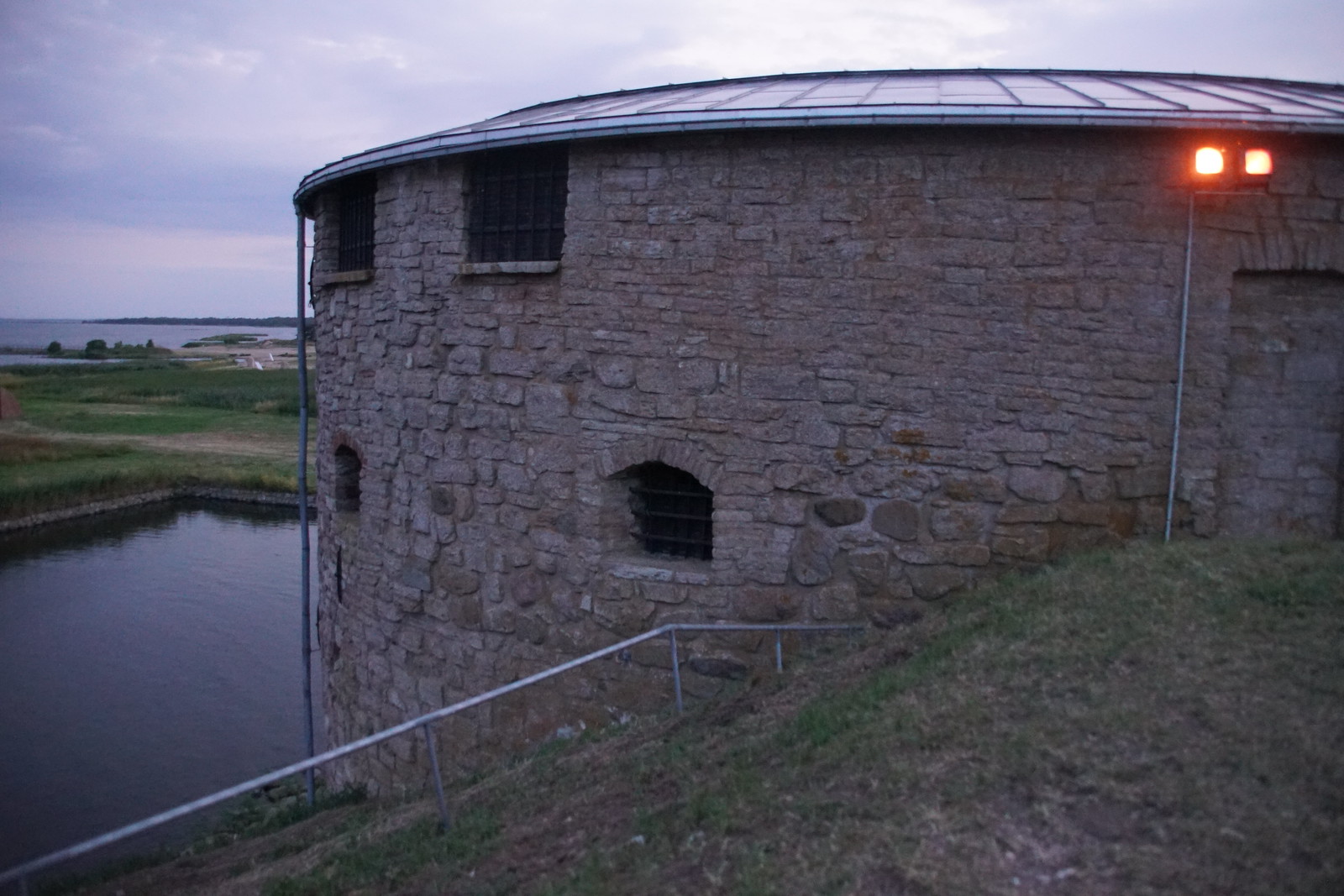The photograph, taken towards dusk, features an old, large circular stone building that resembles a water treatment plant or a pump house. The building, constructed from brick or stone, has a metal or wood paneled roof. Positioned on the upper right corner of the structure are two orange lights, adding a distinct glow to the scene. The building is characterized by several window openings, with some featuring iron bars. Adjacent to the building on the lower left side is a square, flat-surfaced man-made reservoir with a small silver railing overlooking the water. Beyond this artificial reservoir, the background transitions into a field with greenery and a dirt road, eventually leading to a larger body of water, possibly a bay or part of an ocean. The sky is filled with clouds, casting a bluish-purplish hue over the entire landscape.